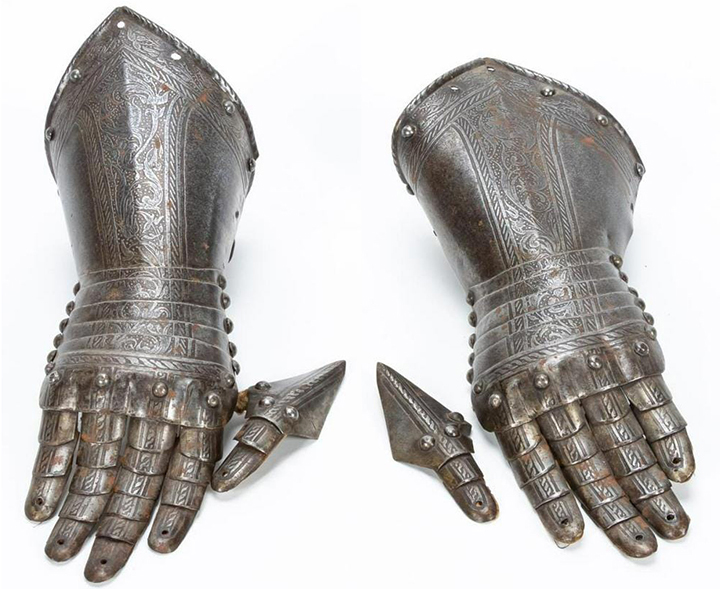This photograph depicts a pair of medieval gauntlets laid out on a white surface. These intricately designed metal gloves are part of a suit of armor and cover the hands and forearms. The gauntlets are made of silver-gray steel, showing signs of rust on some finger joints. The metal includes rivets distributed along the knuckles, the upper forearm area, and the side of the hands, indicating a sturdy construction meant for combat. The fingers appear to be flexible with multiple articulating points, and the detached thumb covers sit adjacent to the main gloves. Ornate filigree decorations, resembling vine patterns, adorn the top center of the gauntlets, adding to their decorative and historical appeal. Accompanied by these are two arrow-shaped accessories positioned between the gauntlets, made of the same gray steel with similar rivet detailing.